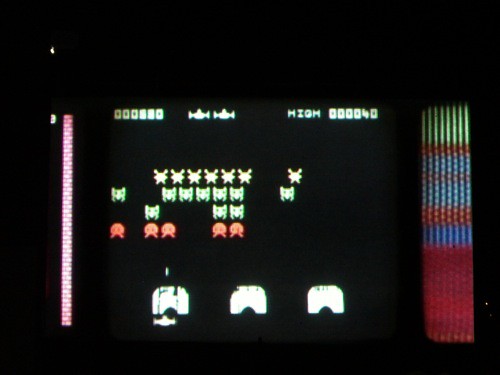This image showcases the classic arcade game Galaga, captured mid-game in an old large arcade cabinet from the 1980s. The scene is bathed in a very dark background that accentuates the screen, making its vibrant details stand out. On the screen, a small white spaceship at the bottom is fiercely shooting upwards at a formation of pixelated, colorful aliens descending from above. The first row of enemies features five red aliens with two eyestalks and tentacles, hinting at their menacing advance. Behind them, a dozen or so light green, crab-like aliens with pincers move steadily downward. At the very top, a row of white rabbit-like aliens adds to the complexity of the assault. The edges of the screen are adorned with a colorful array of borders: a pink bar on one side and a multi-colored strip consisting of red, blue, and green hues on the other. The game’s high score, displayed at the top, is a mere 40, indicating the game has just begun. The current score reads 80, hinting at the player's early progress, while two remaining lives are also visible on the display.